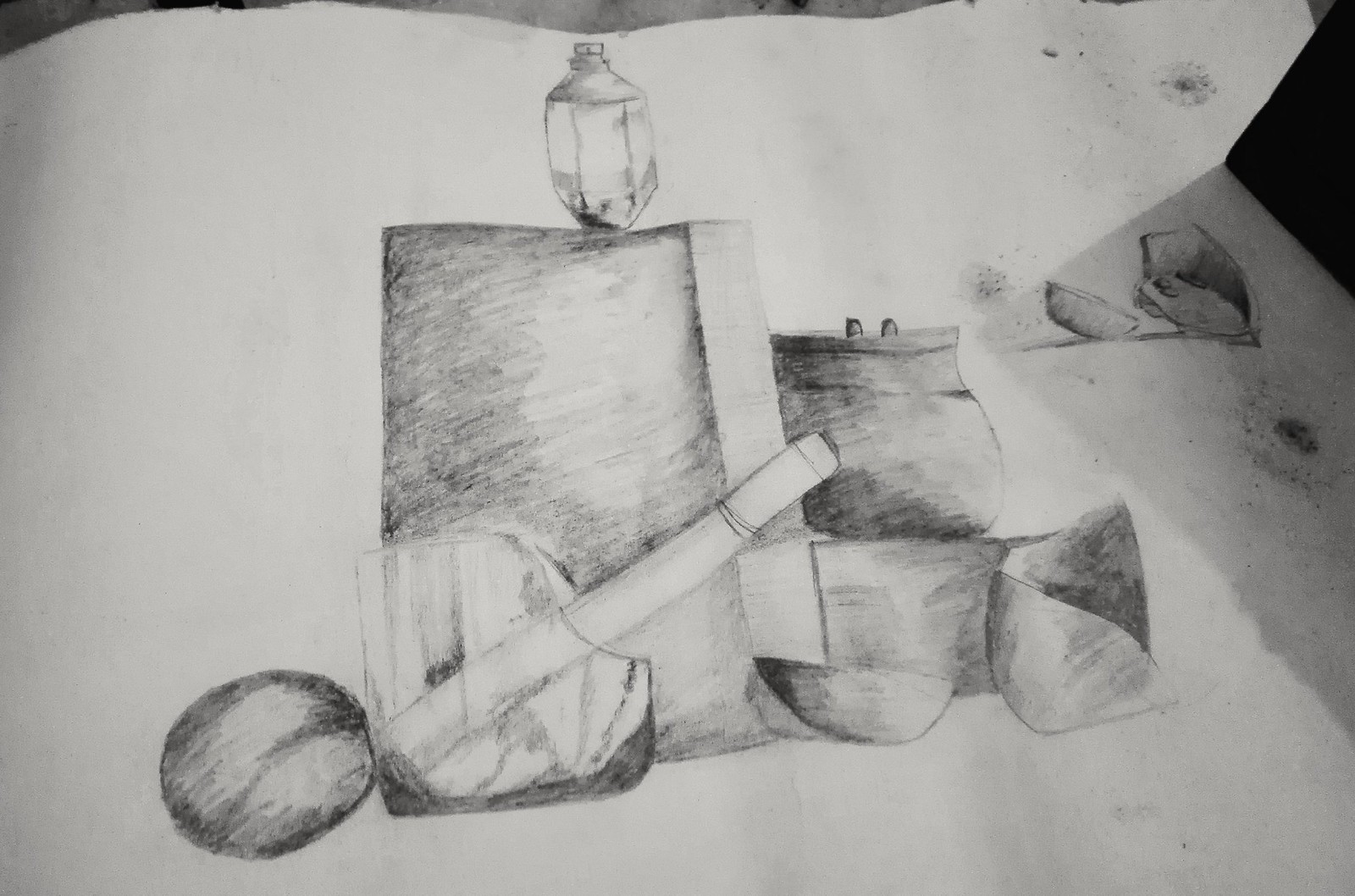This detailed pencil drawing is on a large white sheet of paper. On the far left side of the image is a shaded circle, followed by an object that appears to be a hollow container. Within this container is a cylindrical shape. To the right of this container is a large square shape with a structure that extends downward and curls up at the end. On top of this square shape sits a pot with a lid. Above the pot, there is what seems to be a light or lantern perched on top. On the right side of the drawing, there are a couple of additional images that are indistinguishable.